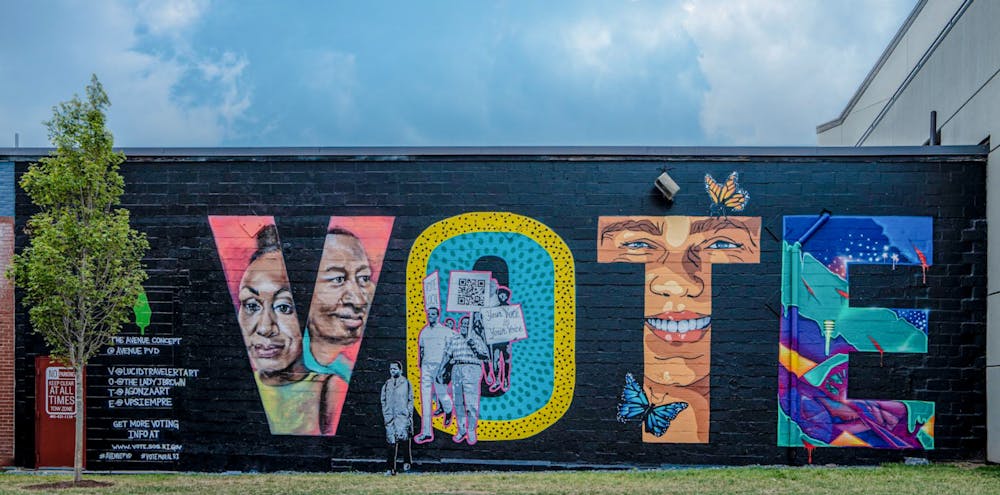In this vibrant mural set against a black brick wall, the word "VOTE" is prominently displayed in large, colorful letters, each harboring unique designs and powerful imagery. The letter "V" features a light peach background adorned with the faces of a black woman and a black man. The "O" contrasts with a yellow-bordered exterior and a teal interior, depicting people protesting with various signs. The "T" showcases a smiling face accompanied by a blue butterfly and a Monarch butterfly. Finally, the "E" invokes the Statue of Liberty with its copper-green hues, featuring a torch and a night sky backdrop. 

The mural, attributed to several artists—Lucid Traveler Tart for the "V," Lady J. Brown for the "O," Agans Art for the "T," and Upsy Empire for the "E"—also features inscriptions about voting information. Trees and the city skyline serve as background elements, enhancing the mural's urban setting and integrating with the overall theme of civic engagement.